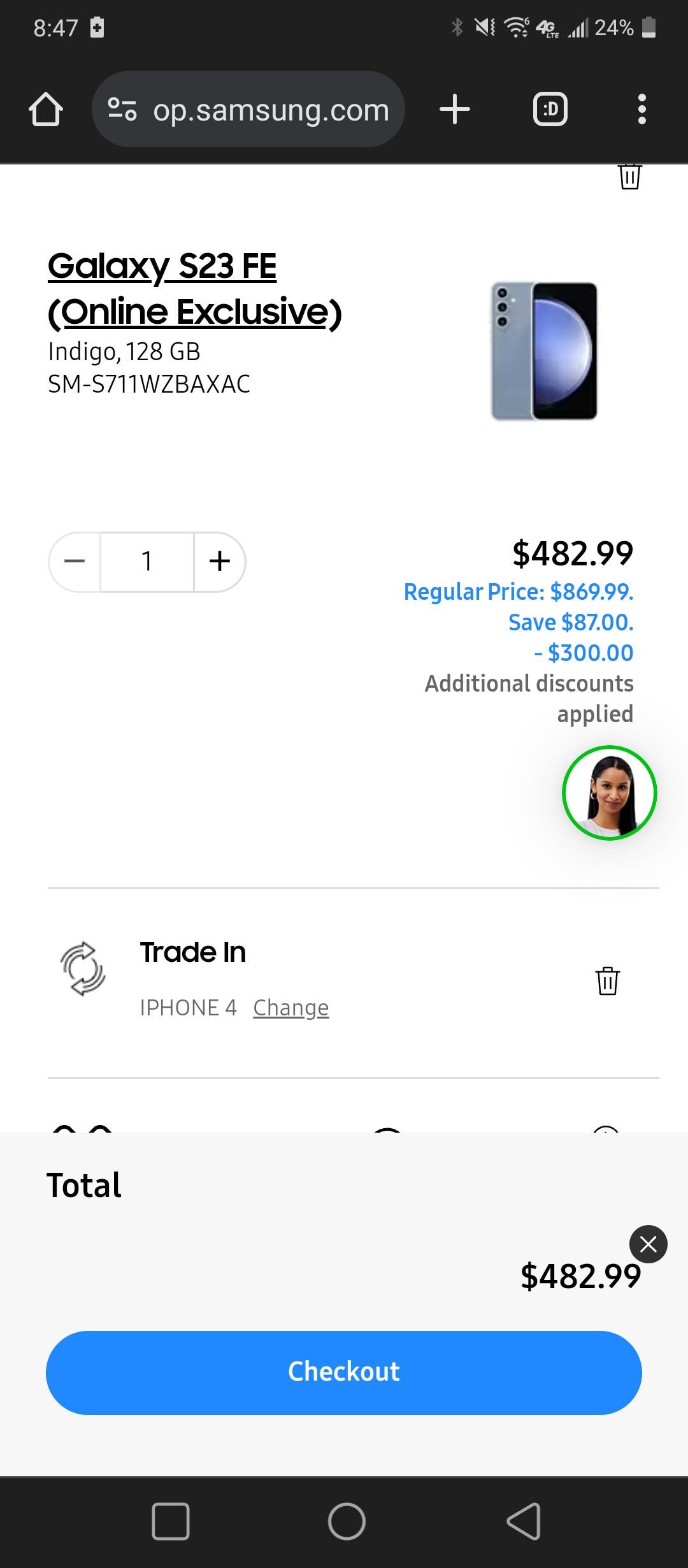This is a highly detailed screenshot captured from a mobile phone, showcasing the Samsung website's product page for purchasing the Galaxy S23 FE Online Exclusive smartphone. Set against a clean, white background, the product title "Samsung Galaxy S23 FE Online Exclusive" is prominently displayed in bold black text. 

To the right of this title, there are two high-resolution images of the phone: one depicting the front and the other the back of the device. The back of the phone is a sleek silver color and features three vertically aligned cameras. The front display exhibits a captivating palette of black and blue tones. 

Below the images, specific product details are listed: "Indigo 128GB SM-S711WZBAXAC." 

The phone is priced at $482.99. Towards the bottom of the screenshot, there's a conspicuous blue oval button labeled "Checkout," accompanied by the total price of $482.99 directly above it. 

Additionally, a small circular icon containing a girl's face is visible below the listed price.